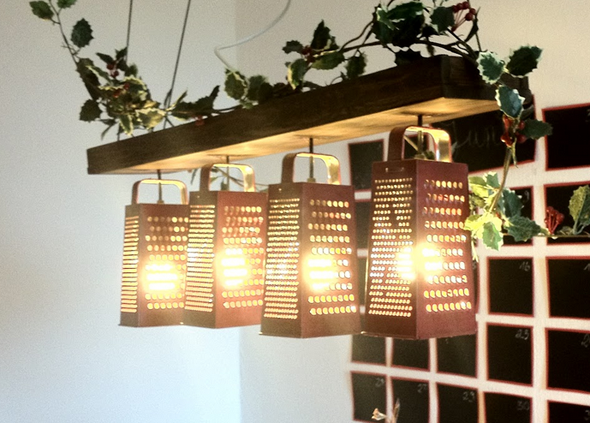This is a color photograph of a unique, homemade hanging light fixture, prominently featured in a room with stark white walls and a window with multiple small panes in the background. The top of the fixture is a solid rectangular block, possibly black, about two to three feet long, and suspended from the ceiling by four chains. The fixture is accented with ivy or similar foliage that extends from the left, across the top, and down the right side. Hanging from this block are four cheese graters, repurposed as lampshades. Each grater has an incandescent light bulb inside, glowing brightly and casting light through their perforations. The graters, which appear to be either brown or dark gray, are oriented with larger openings on the right side, and smaller openings on the side facing the viewer. The scene captures an innovative blend of rustic and functional design elements, set against the dark night visible through the window.